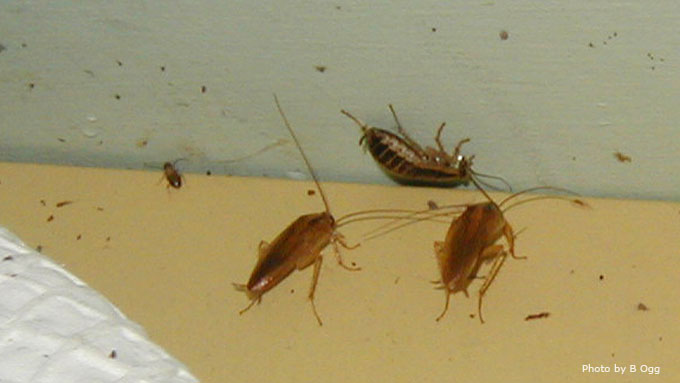This highly detailed image captures a close-up scene of four cockroaches atop a wooden platform on a counter, surrounded by an unsettling amount of dark, brownish droppings. The photograph, marked with a white text watermark reading "Photo by B. Aug" in the bottom-right corner, reveals one cockroach lying upside down, seemingly dead, while two others with long antennas—longer than their bodies—approach it, possibly inspecting or curious. A smaller roach is visible on the left side, staying still amidst the filth. To the bottom-right, a piece of white cloth or textured material, possibly a napkin or pillow, adds to the cluttered and unhygienic scene, while a gray wall with a tan trim forms the background, enhancing the overall dismal atmosphere.